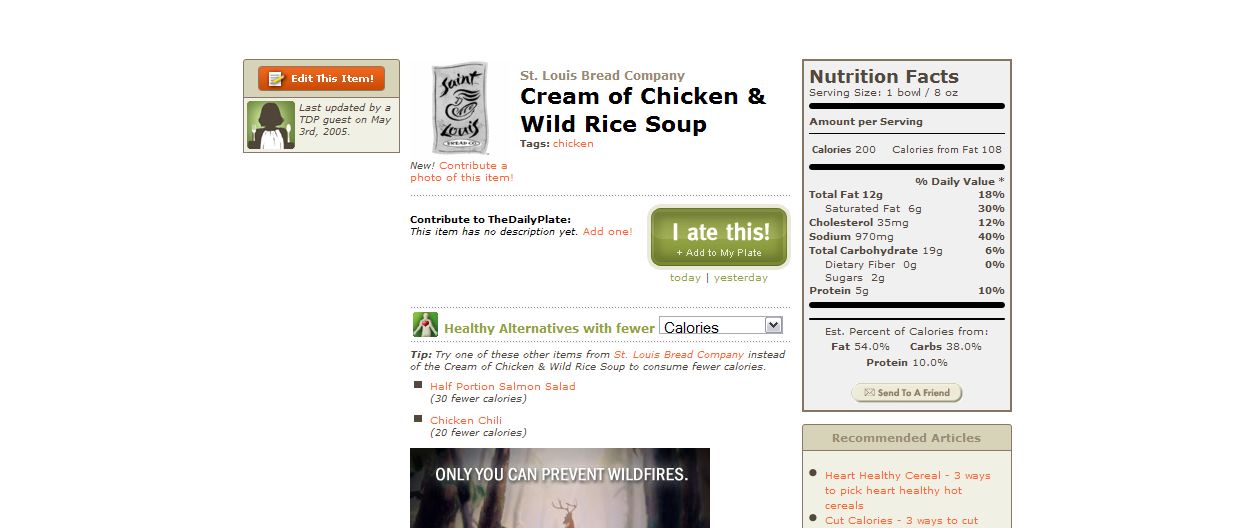This screenshot captures a detailed webpage from the Daily Plate, focusing on a recipe for Cream of Chicken and Wild Rice Soup from the St. Louis Bread Company. At the top, the page prominently displays "St. Louis Bread Company" with a small logo to the left of the title. The recipe name, "Cream of Chicken and Wild Rice Soup," is followed by a tag labeled "chicken" and a "new" tag. There's a prompt below inviting users to "contribute a photo of this item."

The webpage provides nutritional facts in a clearly defined rectangular box on the right-hand side. The specifics include a serving size of 1 bowl (8 ounces), with 200 calories per serving, 108 of which are from fat. The total fat content is 12 grams (18% of daily value), saturated fat at 6 grams (30%), cholesterol at 35 milligrams (12%), sodium at 970 milligrams (40%), total carbohydrates at 19 grams (6%), dietary fiber at 0 grams (0%), sugars at 2 grams, and protein at 5 grams (10%). An estimated percentage chart shows calories from fat at 54%, carbs at 38%, and protein at 10%.

Below the nutritional facts, there is a "send to a friend" option. Additionally, recommended articles are briefly mentioned underneath, including topics like heart-healthy cereals and calorie-cutting tips, though some parts of the text are cut off. To the left of the recommended articles, there is a partial ad, featuring a message about wildfire prevention.

The left panel of the page has options to interact with the recipe, including a button labeled "I ate this" and another prompt encouraging users to add to their daily plate due to the lack of an existing description. There's also a section suggesting healthier alternatives, such as a half portion salmon salad (30 fewer calories) and chicken chili (24 fewer calories). 

Lastly, on the top left side of the webpage, there's an "edit this item" button indicating the last update was made by a TDP guest on May 3, 2005, which hints at some sort of forum-based interactivity on the site.